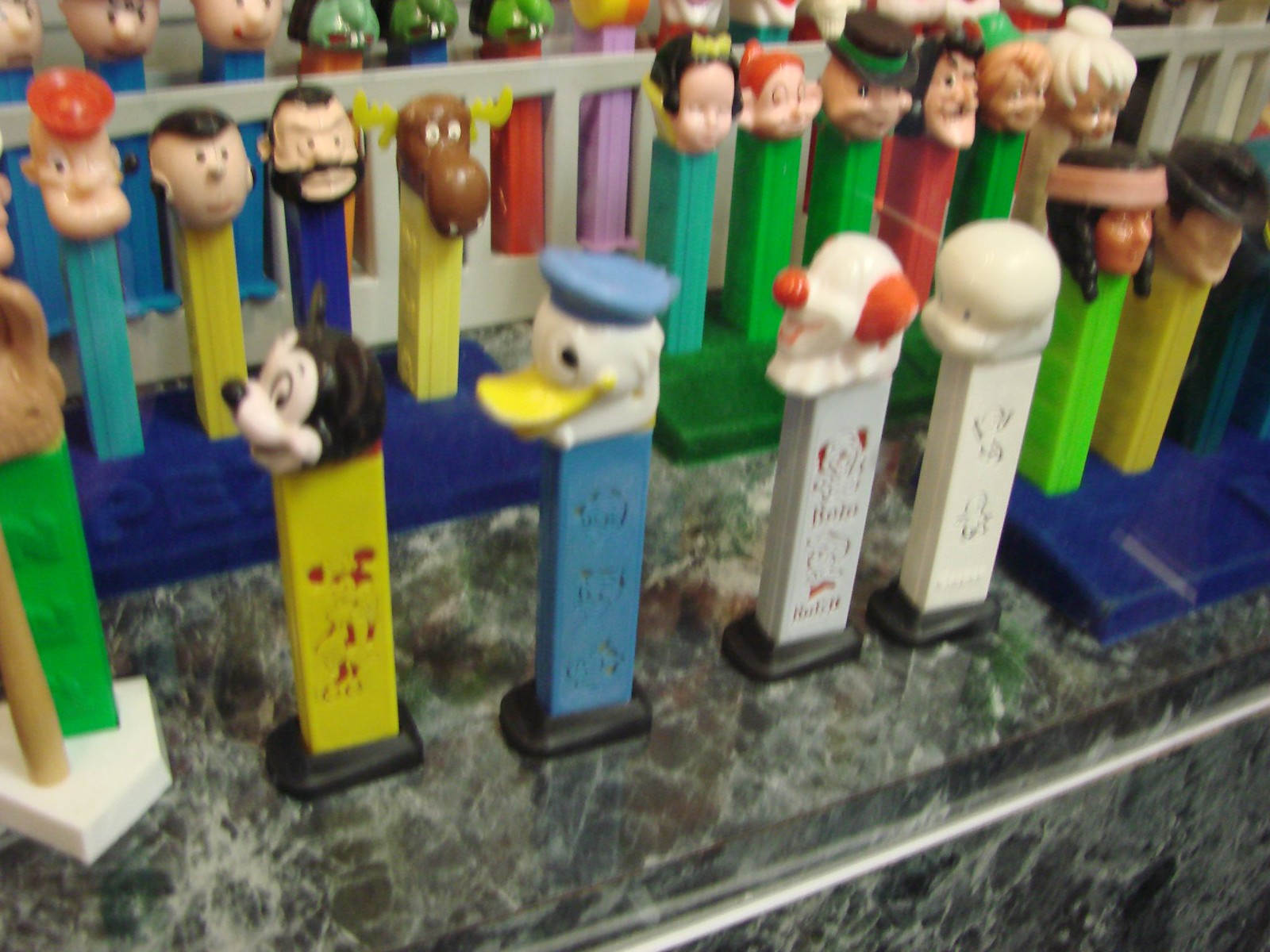In this somewhat faded and blurry full-color indoor photograph, a collection of vintage Pez dispensers is displayed on a marble or faux marble countertop. The dispensers are organized into three diagonal rows, extending from the front lower corner to the upper right corner of the image. The collection features a mix of well-known and obscure characters, likely dating back to the 1970s.

In the front row, you can clearly see a green dispenser with a brown head, possibly referencing a baseball theme, a yellow Mickey Mouse dispenser, and a blue Donald Duck dispenser. Next to these are two white dispensers: one resembling Casper the Ghost, and another with a red nose and red hair. To the right, there's a green Native American-themed dispenser standing beside a park ranger.

The middle row showcases various characters, including Popeye, Olive Oyl, Rocky and Bullwinkle, and Snow White. The back row comprises dispensers with a mix of blue and green faces, with some characters like Pebbles from The Flintstones.

These Pez dispensers, with their spring-loaded heads, were not only used to dispense candy but also served as playful memorabilia, evoking a sense of nostalgia and childhood memories.